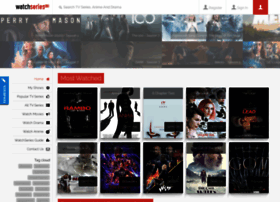The image depicts a webpage interface designed for streaming TV shows and movies. Though the image is small and details are difficult to discern, the primary layout can be described as follows:

At the top of the page, there's a white navigation bar. On the far left, a label reads "Watch Series," with "Watch" written in black and "Series" in red. Adjacent to this label, there appears to be a search bar, followed by two icons that likely represent options to log in or register. Further to the right is another icon accompanied by a red button, though the icon's specifics are unclear.

Below the navigation bar, the main content area displays a selection of movie and TV show titles. This section seems to serve as a showcase for the platform's available offerings. Notable titles visible include "Game of Thrones," a movie featuring Tom Hanks, "The Avengers," and possibly "Black Widow." Another title, which appears to be "The Crow," is also distinguishable.

Underneath this marquee section, there's a red box containing white text, but the text is too small to be legible.

On the left side of the page, there is a vertical menu bar with around ten different selectable options, offering navigation and filter choices for the user to explore the various media content.